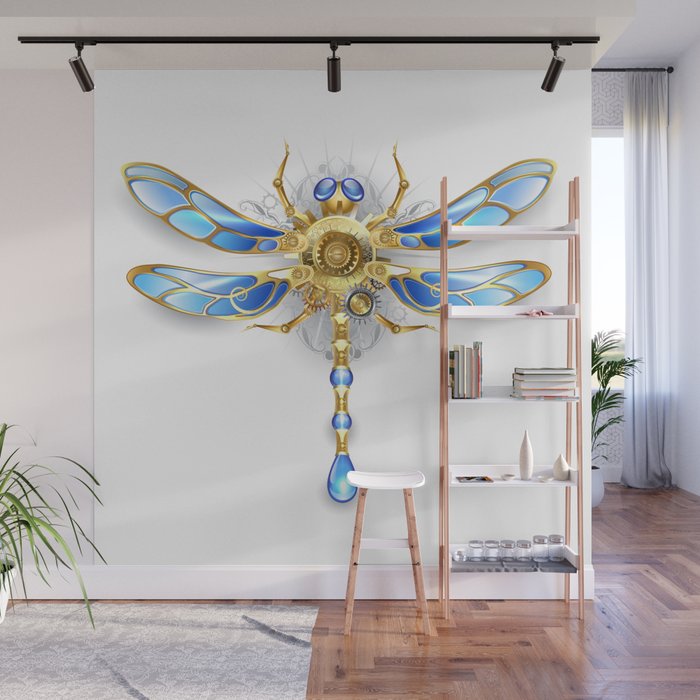This color photograph captures a serene, minimalistic living room with meticulous detail and comforting ambiance. Dominating the white wall is a futuristic, steampunk-inspired dragonfly illustration, displayed on a hanging tapestry. The dragonfly features intricate blue and light blue wings trimmed in gold, a circular gold design at its center, two prominent blue eyes, and a long, slender body adorned with alternating blue and gold dots. The dragonfly's hands are lifted above its head, and it has four wings rather than the typical two.

Above the artwork, three black track lights are positioned but not illuminated, directing attention to the dragonfly. In front of the tapestry stands a ladder-style bookshelf with five rungs, housing books, vases, and glassware of varying sizes and shapes. To the left of the shelf is a wooden stool with a white, oval-shaped seat. The room features a wooden floor, adding warmth to the modern design.

To the left, a glimpse of a potted plant with green foliage spilling out of a white pot can be seen, partially out of frame. The background includes white, floor-to-ceiling sheer curtains that allow sunlight to softly filter through, accompanied by another palm-like plant. This impeccably styled space combines artistic elements with functional decor to create a warm, inviting atmosphere.